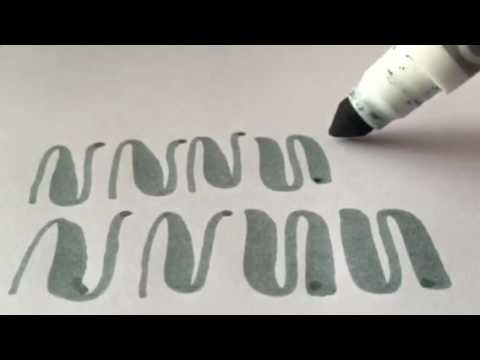The image depicts a piece of light cream-colored paper, bordered by black at the top and bottom edges. A person is using a marker with a light gray barrel and a dark black tip to leave dark gray ink on the paper. The markings appear as random, abstract wave designs that resemble the letter "N" or backward "N" shapes, with fine lines that broaden in sections. These abstract symbols are repeated in a pattern, with four symbols across two rows. The first symbol on the top row and the last two symbols on the bottom row are mirrored. The ink appears somewhat faded, indicating that the marker might be running out of ink and could benefit from being pressed down harder.